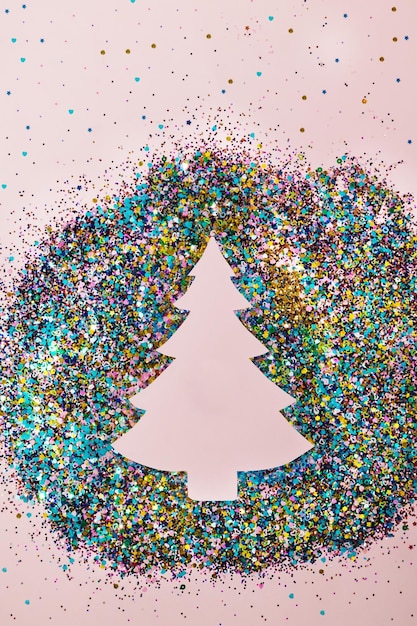The photograph features a cream-colored background with pink undertones, adorned with scattered specks of glitter in blue, gold, and dark green, creating a whimsical, festive atmosphere. Central to the image is a densely packed, multicolored glitter circle comprising shades of turquoise, gold, pink, and white. Within this vibrant circle lies a white cutout of a Christmas tree. Radiating outwards, the glitter forms a sparkling halo around the tree, and the specks of glitter are sparsely scattered across the background, mirroring the top and bottom sections, adding to the overall enchanting and celebratory feel. The intricate details and diverse color palette lend a magical touch to the photograph, highlighting the Christmas tree cutout as the focal point amid a sea of glittering specks.